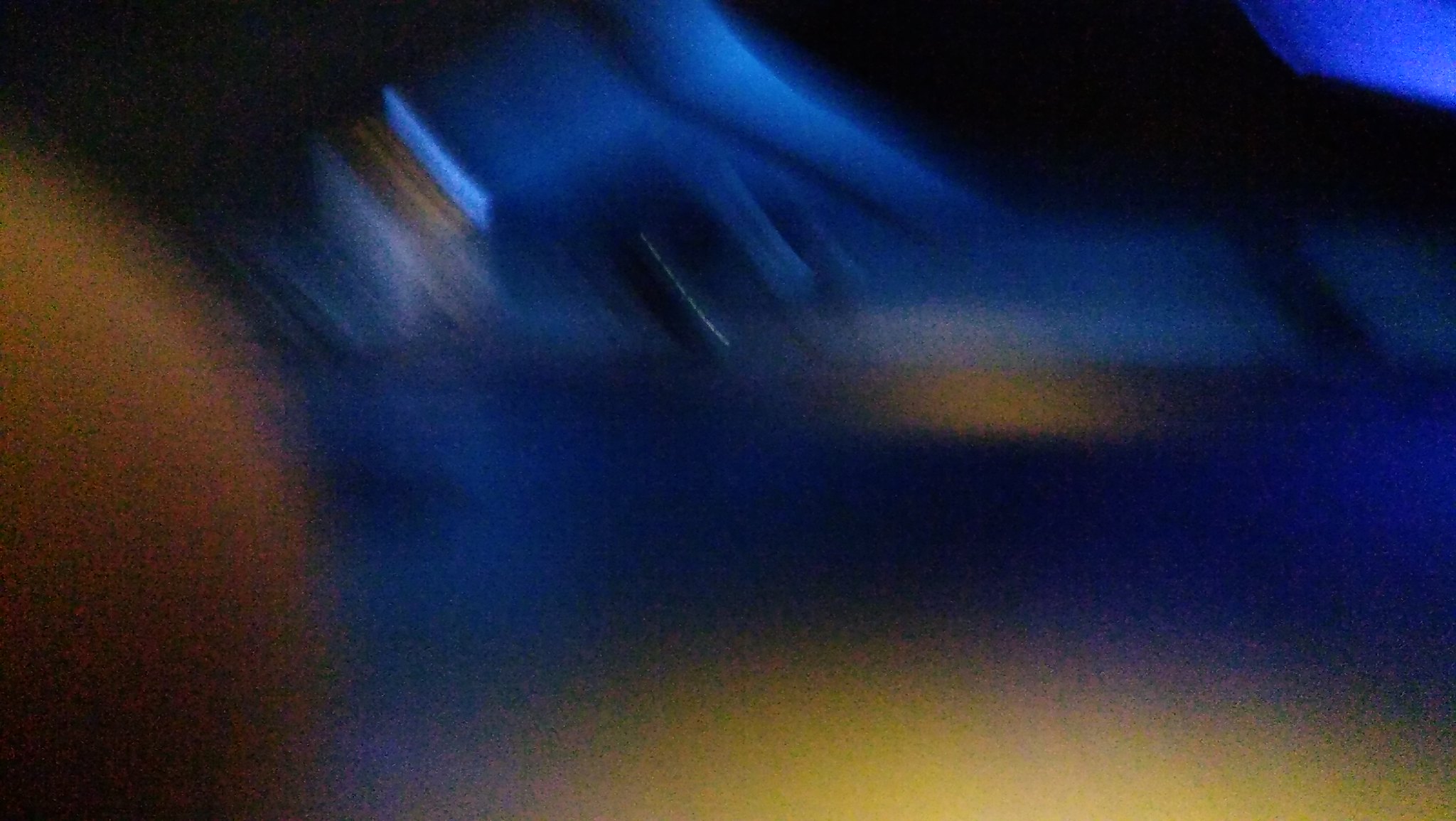A heavily blurred and abstract photograph offers an ambiguous scene with mysterious elements. In the bottom left corner, a brown, vague shape that might resemble the back of a person's head is visible. Centered near the bottom is a round, semi-circular shape, seen from the side. The image is dominated by numerous blue streaks cascading down from above, interspersed with black lines, creating a dynamic yet chaotic pattern. A prominent black mass descends diagonally from the upper left to the mid-right side of the frame. The overall impression suggests a dreamy, imaginative scenario where one might be peering out from within a cave, with the rocky cave roof hovering above and a distant, indistinct view of the sea beyond.